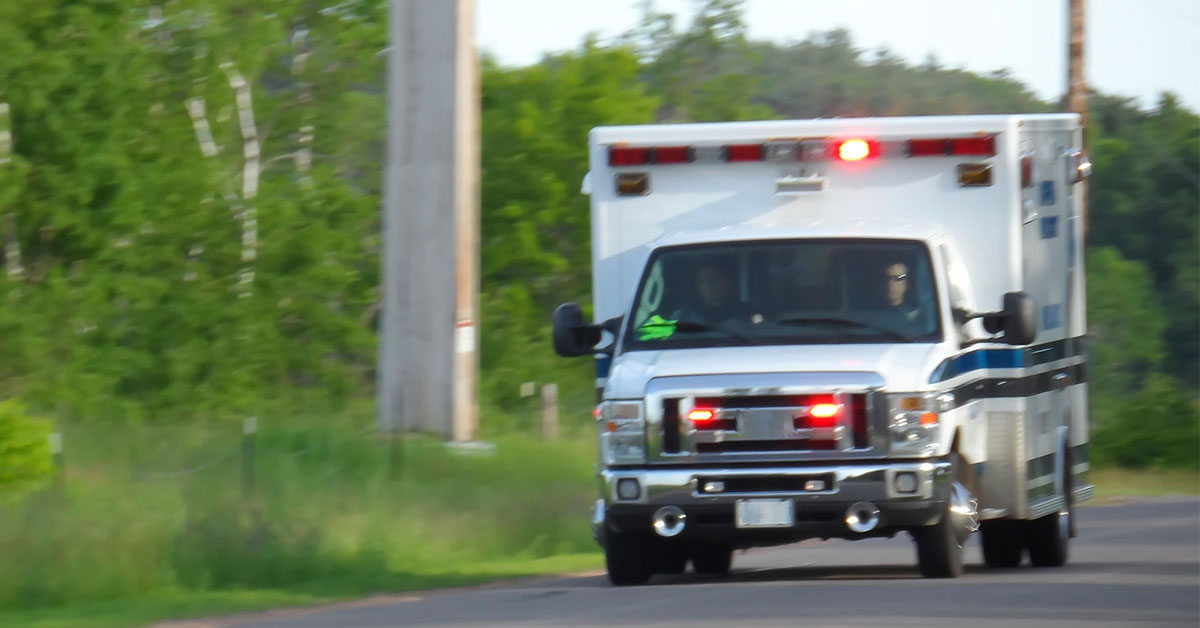This horizontal, rectangular image captures a close-up view of a white ambulance driving down a road, viewed from the front. The photograph, which appears blurry, shows the ambulance with its red and blue lights flashing both on the top and the grill. Blue stripes extend from the driver's side door to the back of the vehicle. The road itself is asphalted and the view includes a bit of it at the bottom, but no other traffic is visible. On the side of the road, there is a grassy area bordered by trees, and a concrete pole that appears to support a large billboard or structure. Inside the ambulance, there are two occupants: the driver, barely discernible and wearing dark glasses, and a male passenger, whose face isn't visible. The image suggests movement, as everything in the scene appears slightly out of focus, potentially taken from a moving vehicle.